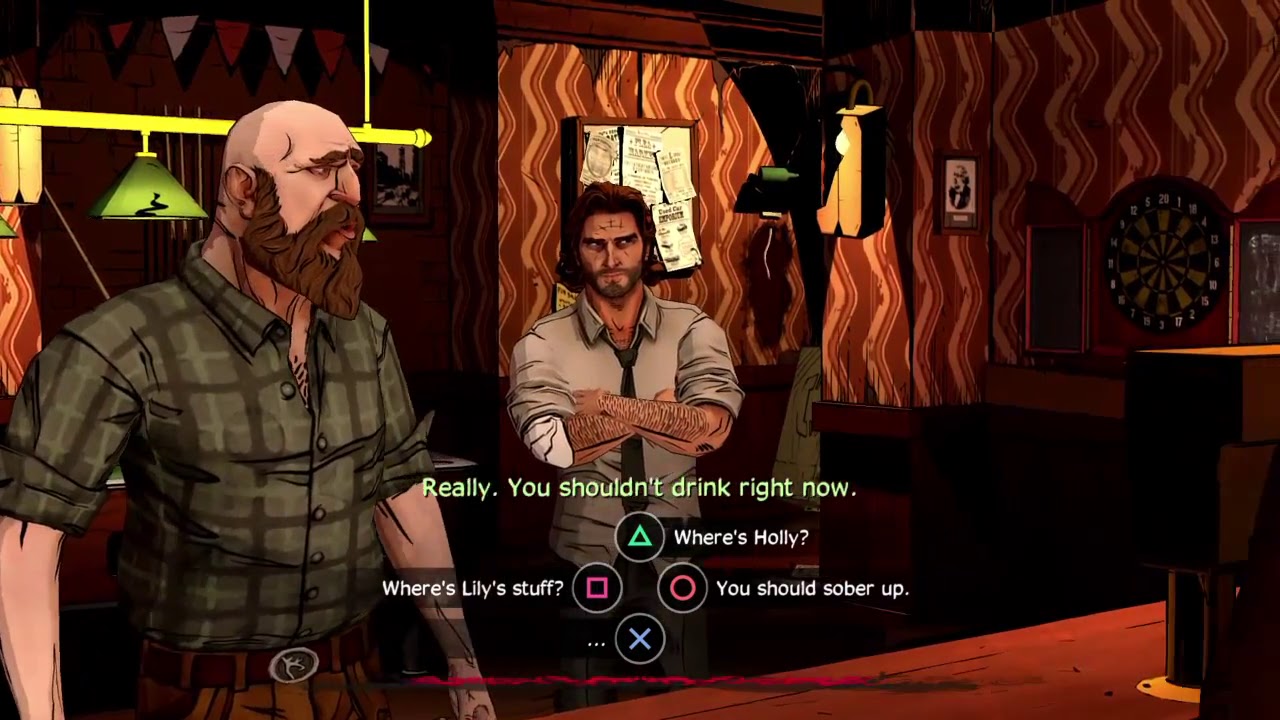In this animated screenshot from a Telltale video game, the scene is set in what appears to be a bar decorated with wavy burgundy and cream-colored wallpaper on the right wall. On this wall, a jagged painting and a dartboard are visible. Near the center, a gold metal bar with green lampshades illuminates a pool table below. The atmosphere is charged with tension as dialogue options are displayed at the bottom of the screen for the player to choose from, indicating an interaction. The text in green letters prompts, "Really? You shouldn't drink right now," followed by options: "Where's Holly?" assigned to the triangle button, "You should sober up," for the circle button, "…" for the X button, and "Where's Lily's stuff?" designated to the square button.

Two distinct male characters occupy the scene. On the left stands a big, bald man with a thick brown beard and mustache, wearing a green plaid shirt with sleeves rolled up to his elbows and brown jeans secured by a silver belt buckle. His attire and appearance suggest a rugged persona. To his right is a white man with long brown hair, a serious expression, and a trimmed beard and mustache. He is dressed in a slightly disheveled white dress shirt, with the collar unbuttoned and sleeves rolled up, showing his hairy arms. He also wears a black tie. Both characters are deeply engrossed in what seems to be a significant conversation, highlighted by the player’s ability to guide the interaction.